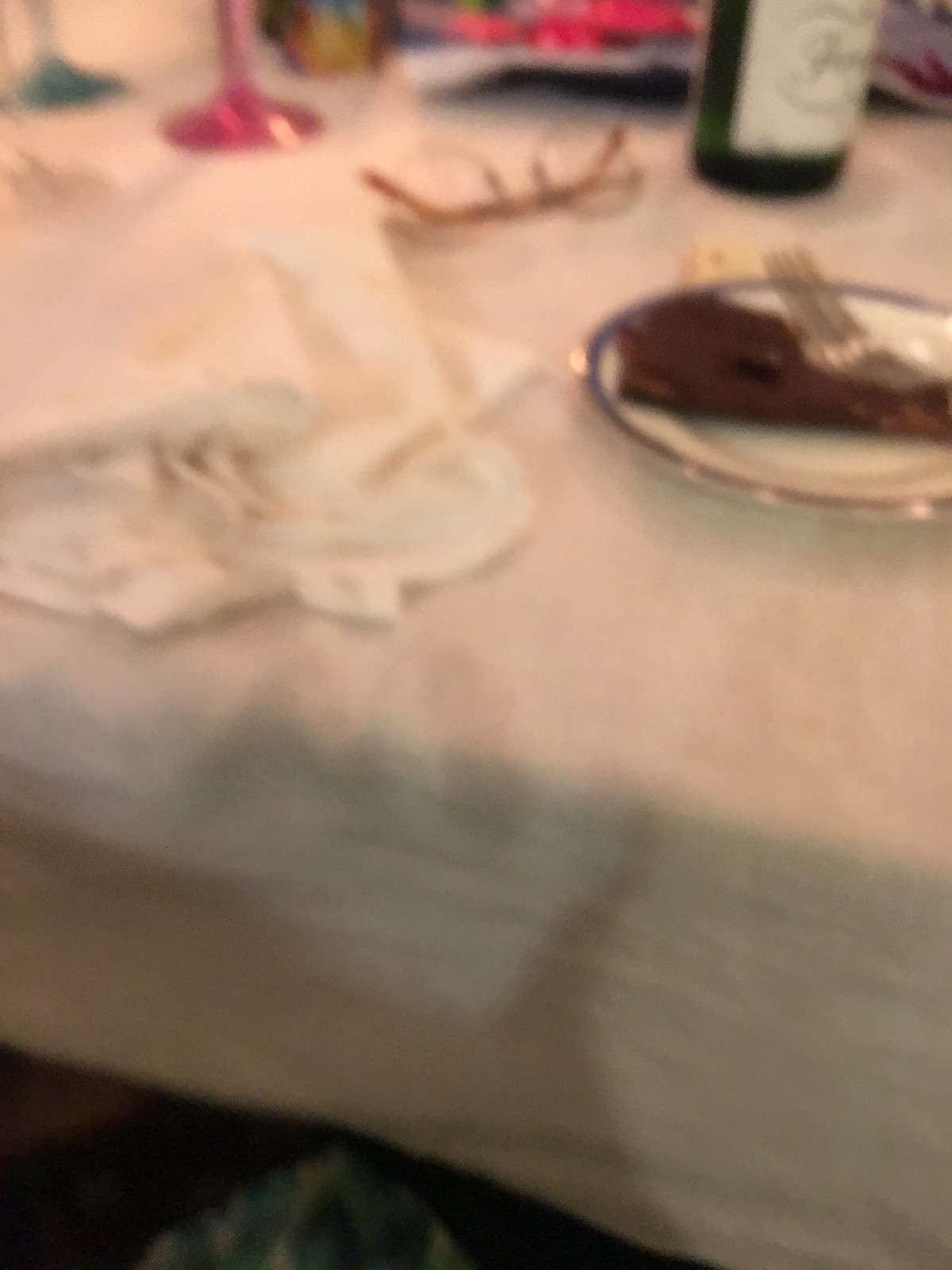This image depicts a close-up shot of a tabletop covered with a white tablecloth. On the right side of the table, there is a white plate adorned with a blue border. Resting on the plate is a silver fork facing upward and a piece of brown food, possibly chocolate cake. Adjacent to the plate on the left is a folded white cloth or napkin. Above the napkin sit a pair of black-framed prescription glasses with clear lenses. To the right of the glasses, there is a green glass bottle featuring a white label that faces to the right. Towards the top of the image sit two wine glasses, one pink and one blue. Additionally, various indistinct colored objects in red, yellow, and green are visible in the blurred background. The white tablecloth drapes down 4 to 5 inches along the side of the table.